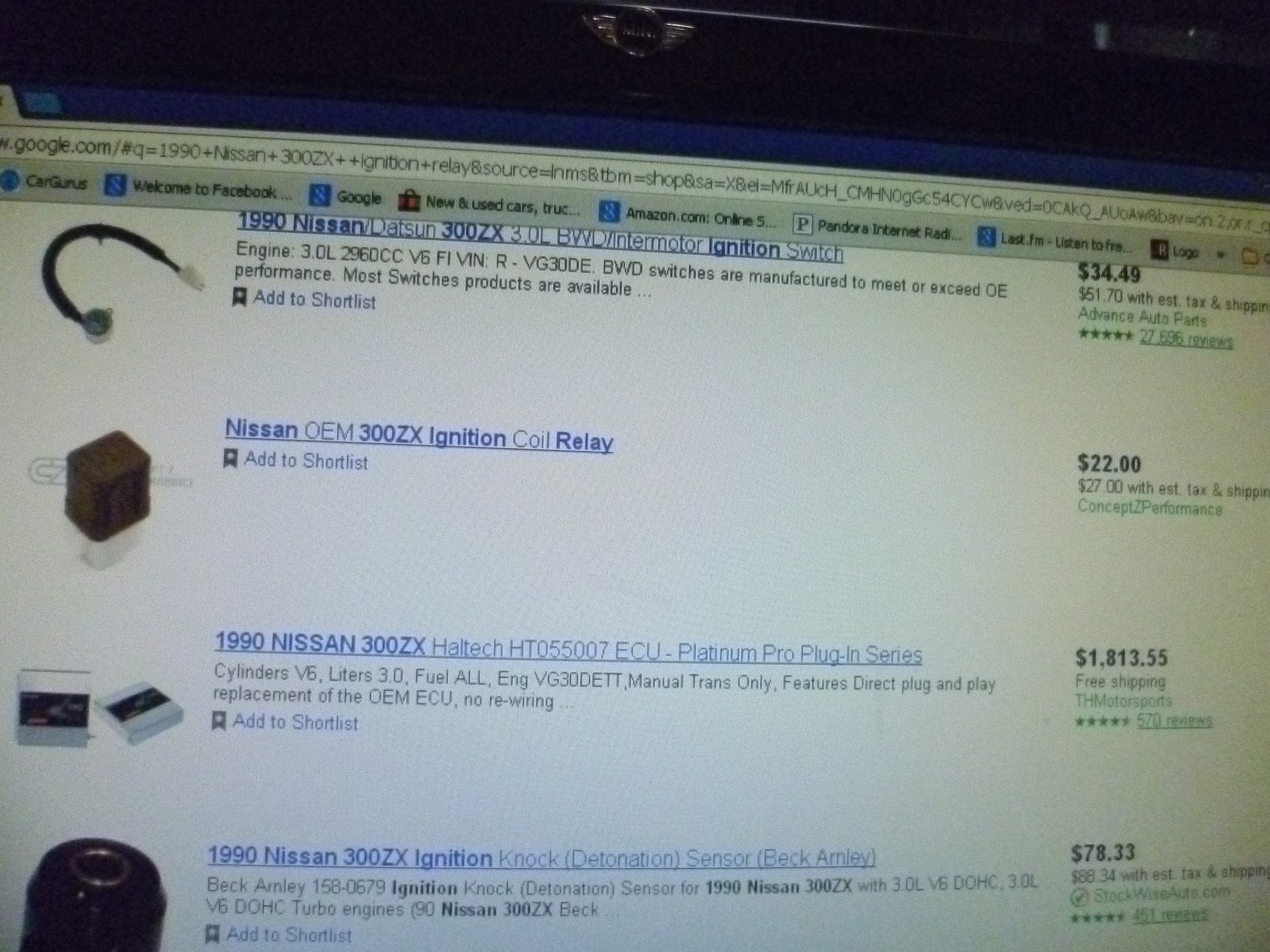This image depicts a Google Shopping page displaying various components for a 1990 Nissan 300ZX. The highlighted products include a 1990 Nissan ignition switch priced at $35, which features a cable connector. Another item is a coil relay, a small electronic box used for controlling electrical circuits. Additionally, an ECU (Electronic Control Unit) is listed with a substantial price tag of $1,800 and offers free shipping. Lastly, an ignition knock sensor is available for $78, identified by its cylindrical shape. All products display inclusive taxes and shipping costs, emphasizing the comprehensive nature of the listings found through Google Shopping.